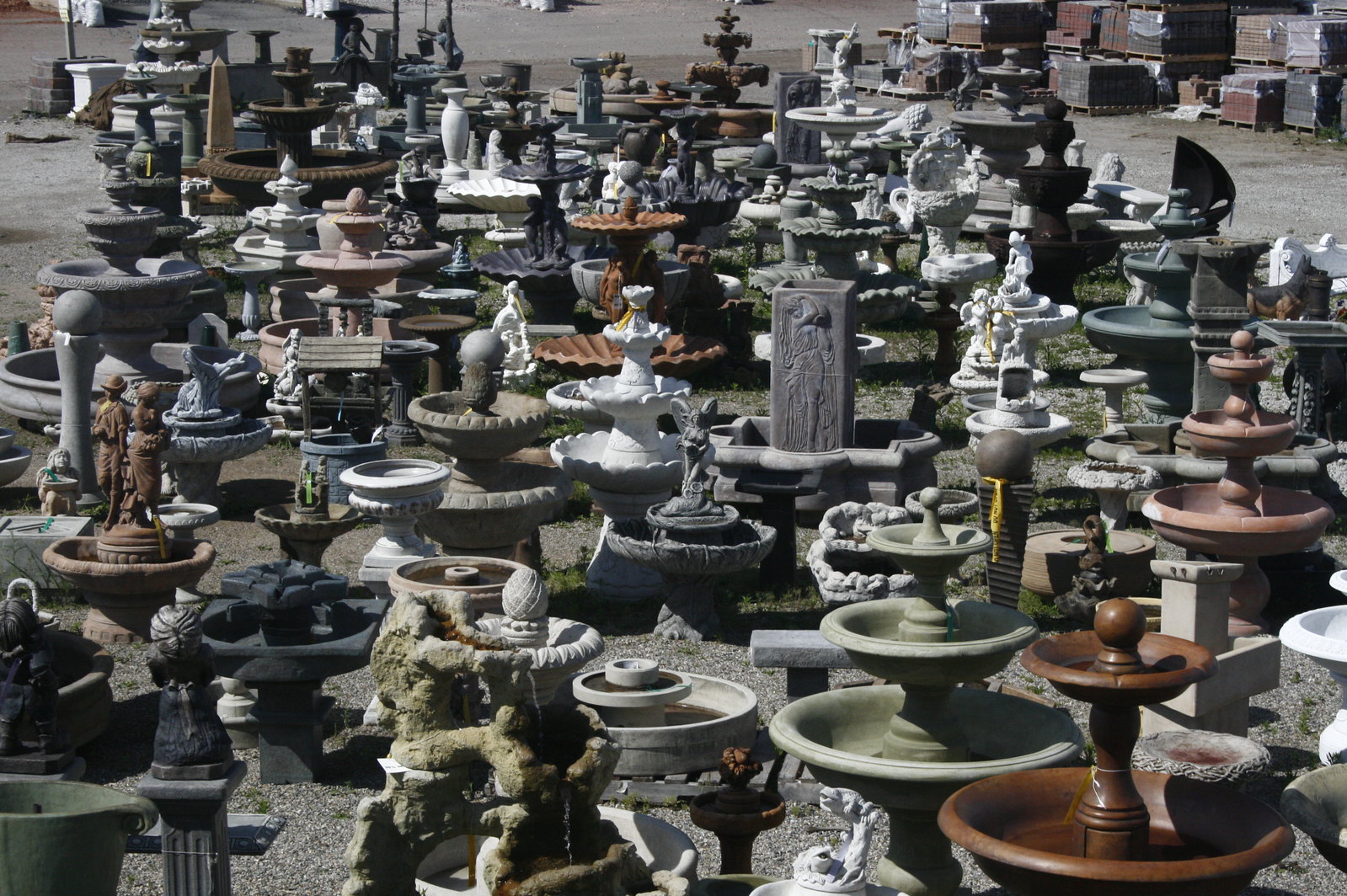The photograph depicts an outdoor setting at what appears to be a garden center, showcasing an extensive collection of garden birdbaths, fountains, and statuary items. These objects are densely arranged on a flat, concrete or gray gravel surface, making it challenging to navigate between them. The items vary in color, including shades of gray, terracotta, white, brown, pink, and mossy green. The fountains and birdbaths exhibit diverse designs, from simple Greek column styles to elaborate multi-tiered pieces adorned with figures like angels and people. None of the water features are filled or active, suggesting they may be for display or sale rather than in use. In the background, assorted cases and crates add to the impression of a commercial garden supply area. The sunlight casts distinct shadows on the ground, highlighting the textures and forms of the numerous items.